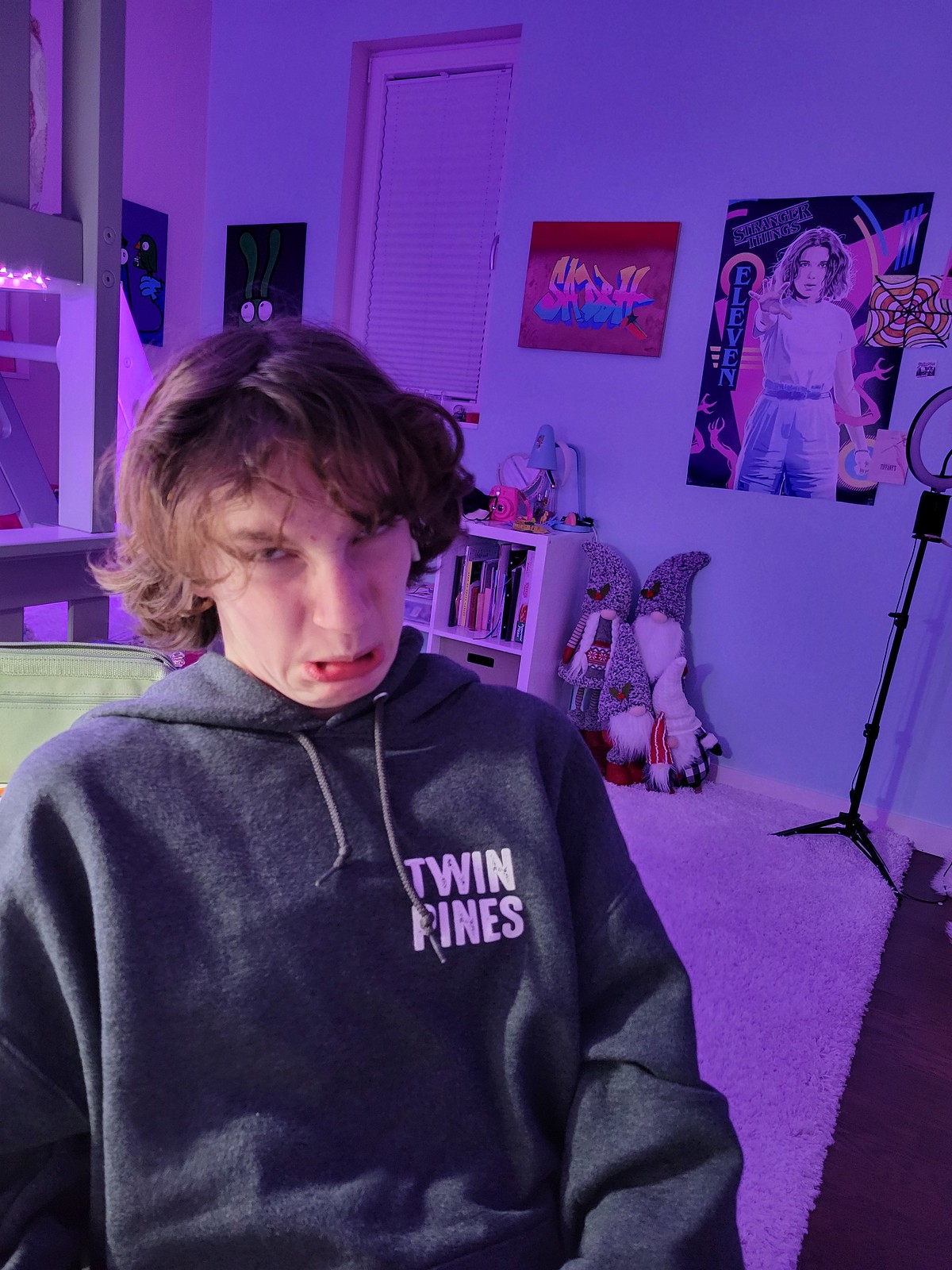In this vertically aligned, somewhat dark image, a teenage boy sits in a dimly lit bedroom, making a silly, unhappy face while looking directly at the camera. He is dressed in a gray drawstring hoodie with the words "Twin Pines" in white text on the left chest area. The room is accentuated by a moody purple and pink glow, likely from LED lights hidden from view, which casts colored hues onto the carpet and walls. 

The room features several objects and decor: 

- A carpeted floor, partially contrasted by hardwood
- White baseboards lining the walls
- A black ring light stand, partially visible on the right side, placed on the rug
- Two windows, one with visible hanging lights and another with closed blinds
- Wall art and posters, including a prominent one of Eleven from Stranger Things
- A few stuffed animal gnomes sitting next to a bookshelf
- Shelves holding various objects 
- A bed accompanied by the shading of nighttime

The mixture of purple and pink lighting, combined with the scattered elements and teenage memorabilia, suggests a cozy, adolescent indoor setting.